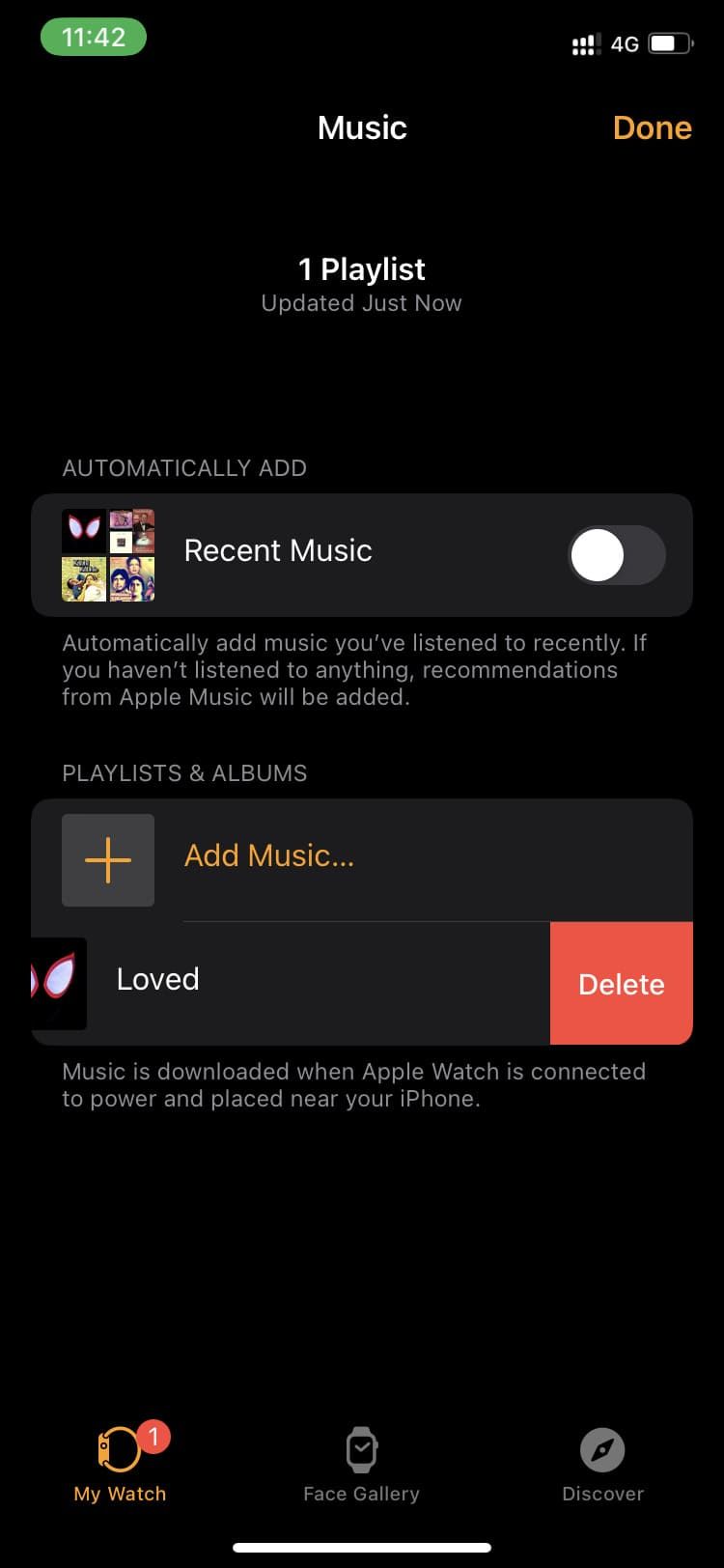This screenshot, taken on a mobile device, has a clean and structured interface against a black background. At the very top-left corner, the time is displayed as "11:42" in green, while the top-right corner shows the 4G network status and a battery icon indicating approximately two-thirds charge. 

The title "Music" is prominently featured in white text at the top, with the word "Done" highlighted in orange on the right-hand side. Below, a notification states “One playlist uploaded just now” in white text, indicating recent activity. 

The section beneath this notification includes an option labeled "Automatically Add," accompanied by a slider currently toggled off. This is followed by the text: "Automatically add music you've listened to recently. If you haven't listened to anything, recommendations from Apple Music will be added." Four album covers are displayed here, denoting recent music.

Further down is a section labeled "Playlists and Albums," featuring a dark gray box with rounded edges. This area has an "Add Music..." prompt in orange text at the top, next to an orange plus sign within a medium gray box. Below this, the word "Loved" appears alongside a partially visible album cover that is primarily black with white and red elements. Adjacent to it is a delete button.

The bottom section states: "Music is downloaded when Apple Watch is connected to power and placed near your iPhone." Lastly, the very bottom edge of the screen displays three navigational icons labeled "My Watch," "Face Gallery," and "Discover."